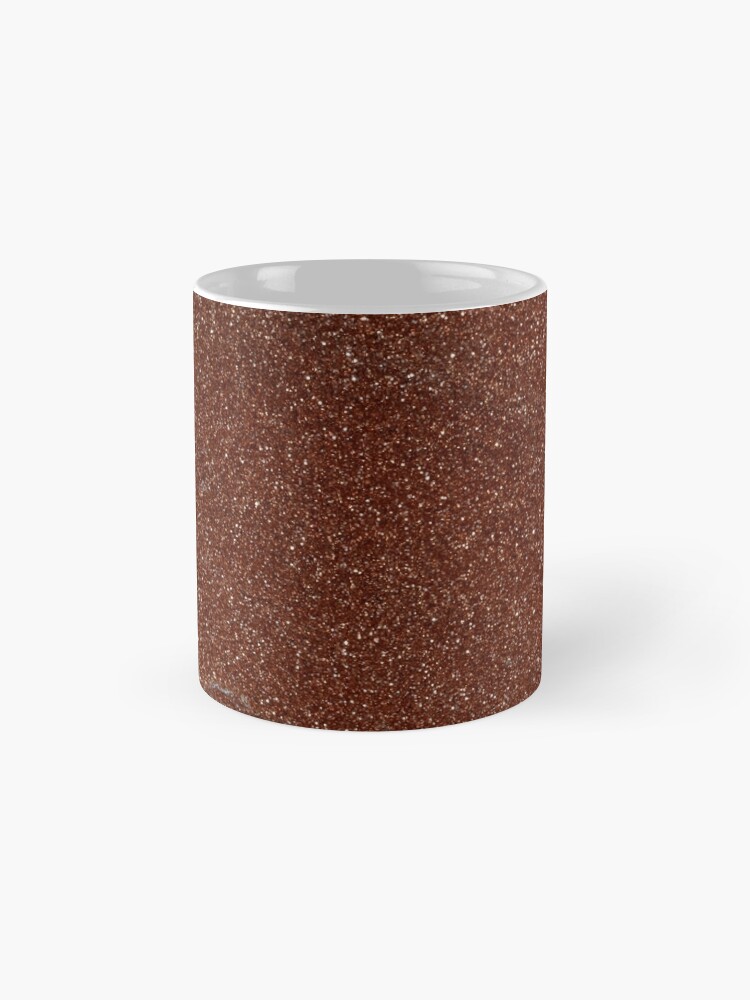The image depicts a professionally taken photograph of a handle-less coffee cup that is centrally positioned against a plain white background, emphasizing simplicity and focus on the cup itself. The cup features a glossy white interior, while its exterior showcases a captivating pattern of burgundy and brown hues interspersed with subtle white speckles. These speckles create a glittery effect, giving the cup a sophisticated sparkle. The pattern varies slightly in shade, with darker tones concentrated at the center and lighter variations towards the edges, likely influenced by the lighting. The cup's design is intricate, suggesting a paisley-like motif formed by the arrangement of the tiny speckles. Despite the seemingly straightforward subject, the detailed patterning and carefully controlled lighting lend the image an air of elegance and artistry.